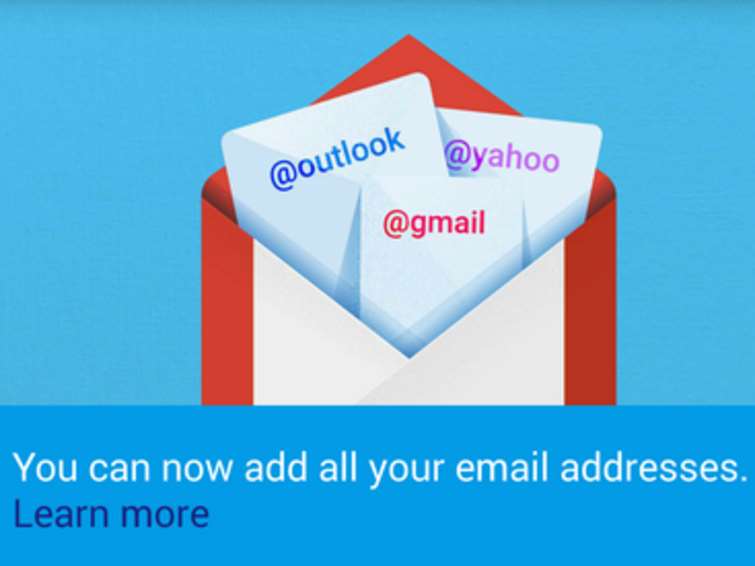This image portrays a stylized envelope resembling the Gmail icon, with a prominent red border and white center. Within this envelope, several email icons, including Outlook, Gmail, and Yahoo, are displayed, symbolizing the integration of multiple email addresses. The backdrop of the image consists of two shades of blue, and the white text across it reads, "Learn how to add all your email addresses," although it is not explicitly clear what kind of account the emails are being linked to. The overall appearance of the image is somewhat low in quality, adding to the ambiguity of its purpose.